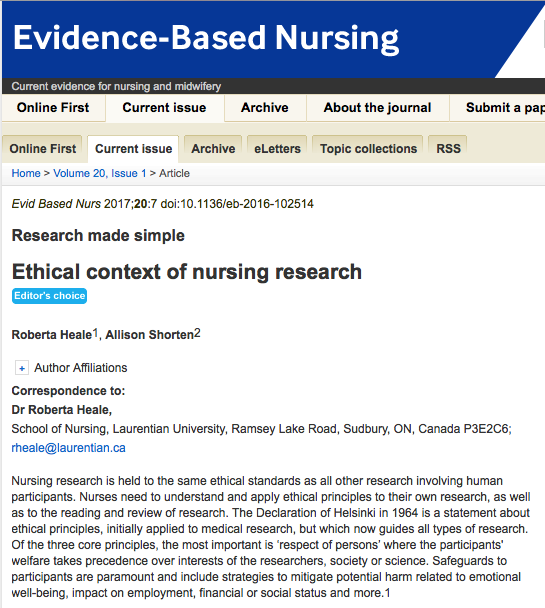The screenshot depicts the top section of a website, highlighted by a blue bar that reads "Evidence-Based Nursing." Below this bar, a header states "Current Evidence for Nursing and Midwifery" with navigation tabs underneath it for "Online First," "Current Issue," "Archive," "About the Journal," "Submit a Paper," although the latter is partially cut off. The active tab shown is "Current Issue," specifically "Home, Volume 20, Issue 1, Article."

The main text on the page is a citation: "EVID-Based NURS 2017, 20(1):207. DOI: 10.1136/EB-2016-102514." The article's title, "Research Made Simple: Ethical Context of Nursing Research," is prominently displayed, labeled as the "Editor's Choice" by Roberta Heal and Allison Shorten. A button is visible to expand the author affiliations. Correspondence information for Dr. Roberta Heal from the School of Nursing at Laurentian University is given, listing her address on Ramsey Lake Road, Sudbury, Ontario, Canada, P3E 2C6, and her email, rheal@laurentian.ca.

The introductory text of the article explains that nursing research adheres to the same ethical standards as other forms of research involving human participants. It emphasizes the necessity for nurses to comprehend and apply these ethical principles in their own research and when evaluating other research. A reference is made to the Declaration of Helsinki established in 1964, which was initially aimed at medical research but has since become a guiding document for all research fields. Among its three core principles, the foremost is respect for persons, ensuring that the welfare of participants surpasses the interests of researchers, society, or science. Essential safeguards include measures to mitigate potential harm affecting participants' emotional well-being, employment status, financial standing, social status, and more.